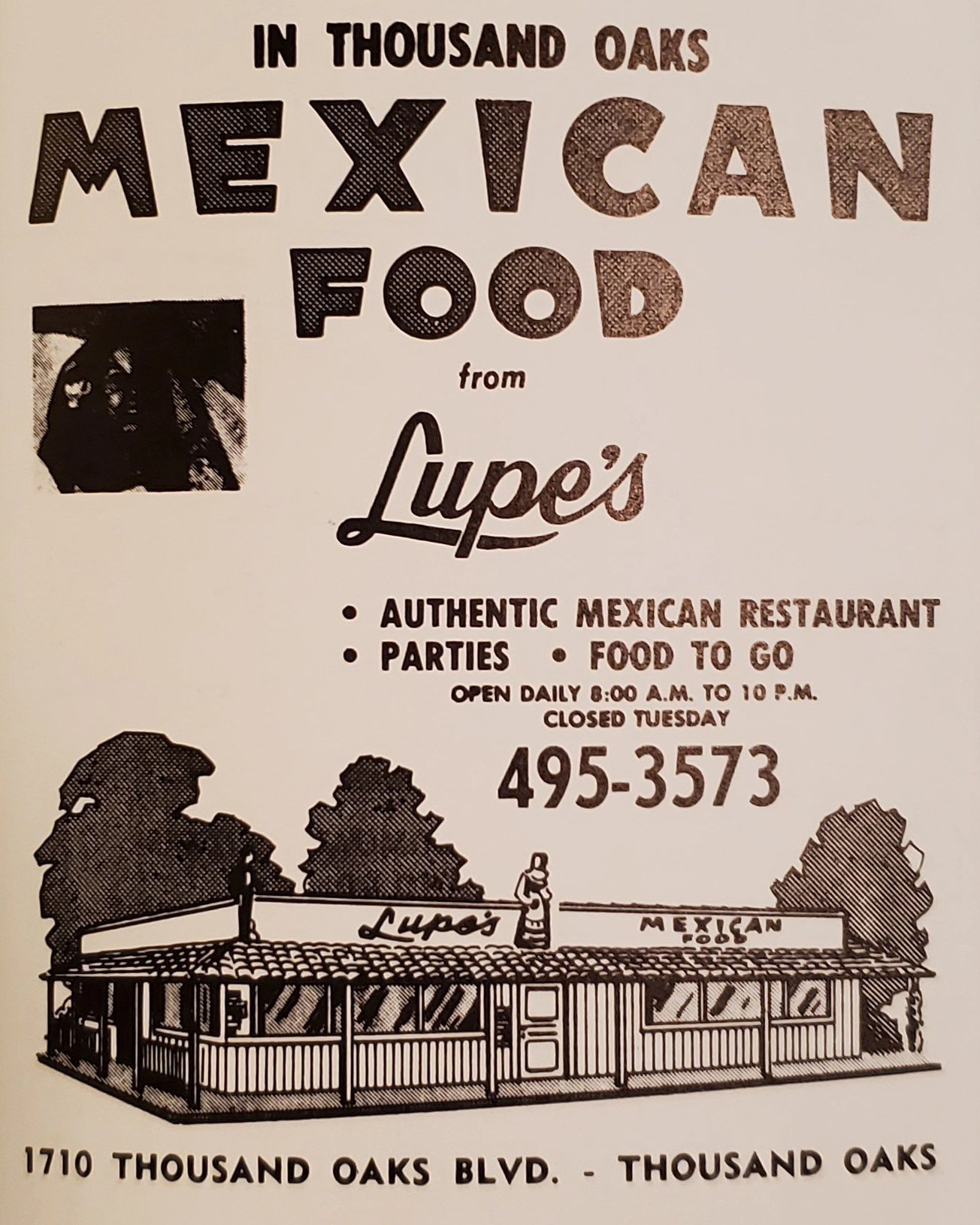This is a black and white illustrated advertisement for Lupe's, a Mexican restaurant located in Thousand Oaks. At the top, large bold letters state "In Thousand Oaks, Mexican Food" with "Lupe's" written in cursive beneath. Below, there are three bullet points: "Authentic Mexican Restaurant," "Parties," and "Food to Go." Further down, it states, "Open Daily, 6 a.m. to 10 p.m. Closed Tuesday" followed by the phone number, "495-3573." At the bottom, the address, "1710 Thousand Oaks Boulevard, Thousand Oaks," is listed. The bottom section features an illustration of the restaurant, a simple one-story building with large windows and an overhanging roof, and three trees in the background. An image of a woman in traditional Mexican dress is located between "Lupe's" and "Mexican Food" at the top right of the advertisement.